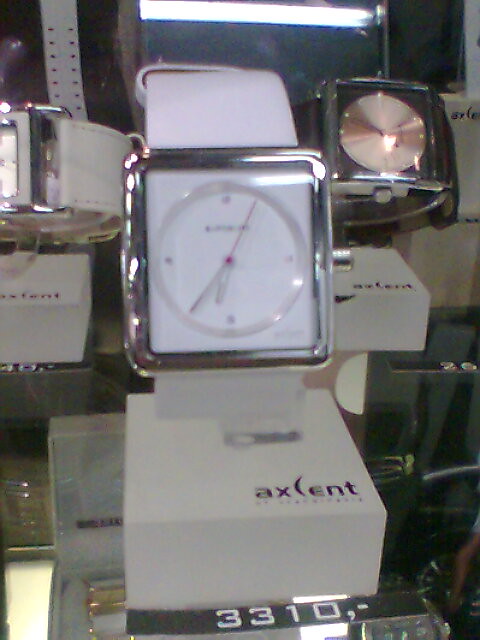This dimly lit and blurry image captures a collection of watches, stacked with their respective boxes. Central to the photo is a prominently featured watch with a shiny square face, encased in a silver rim. The watch face itself is minimalist, adorned with numeric notations only at the 6, 9, 12, and 3 o'clock positions, and the time displayed is 6:40, complete with a second hand. The band of this watch is white and appears to be made of plastic. It is prominently displayed on a cardboard presentation box that reads "X cent." Flanking the central watch are additional timepieces, each resting on their own boxes. Below this primary display, several other watches can be seen, housed within their packaging.